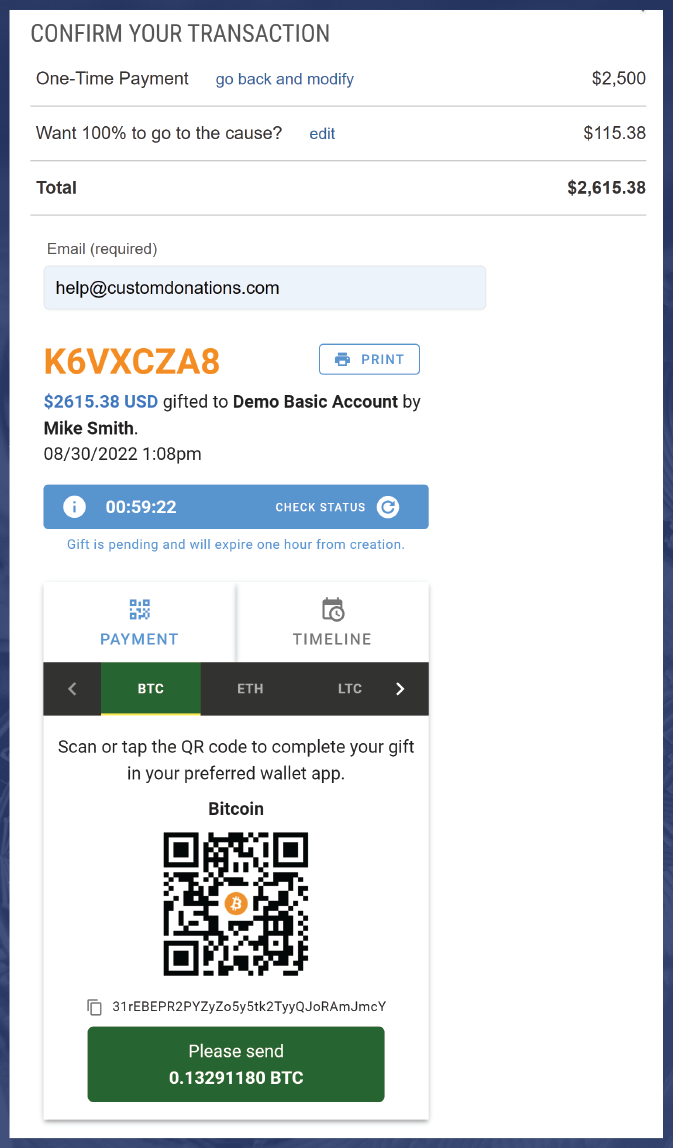This image is a detailed screenshot confirming an order placement. At the top, the heading reads "Confirm Your Transaction." Below, there is a section labeled "One-Time Payment" in black text, adjacent to a blue link that says "Go back and modify," with the amount "$2500" displayed to the far right.

Further down, another section asks, "Want 100% to go to the cause?" accompanied by an interactive blue "Edit" link and the amount "$115.38" below it. 

At the top of the next section, the total amount due is prominently listed as "$2616.38." Below this, an "Email Required" field contains an email address entered into a blue text entry box. Directly below, in large orange letters, is a code "K6VXCZA8," next to which there is a rectangular button labeled "Print."

Centrally located on the image is a timer displaying "59:22" alongside the text "Check Status." Below this, there are two buttons: one for "Payment" and another for "Timeline." 

The lower section of the image features cryptocurrency options, including BTC (Bitcoin), ETH (Ethereum), and LTC (Litecoin), with a central Bitcoin QR code at the bottom. Below the QR code, the instruction reads, "Please send 0.13291180 BTC."